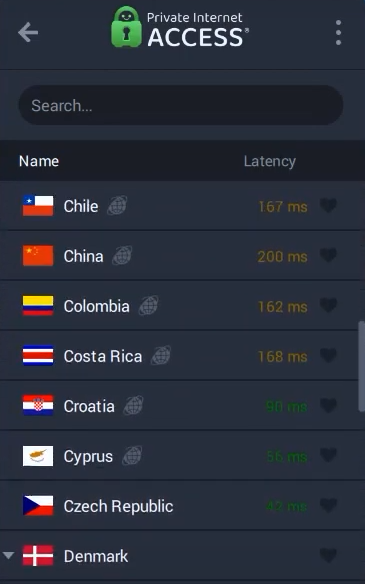This screenshot displays the user interface of the Private Internet Access application.

The background is a deep charcoal black, creating a sleek and modern visual. In the upper left corner, there is a gray directional arrow pointing to the left, likely indicating a back navigation option. Centered prominently, a green padlock icon with a keyhole symbolizes security, followed by the text "Private Internet Access" in clean white font.

In the far upper right corner, three vertical light gray dots suggest more settings or options are available. Just below this, a thin, darker black line stretches horizontally across the screen, dividing the top section from the rest of the interface.

Beneath this line lies a long black search bar with light gray text that reads "Search" on the left side, ending with three more dots.

The next section is a black rectangle divided into two columns by white text. On the left, it reads "Name," and on the right, "Latency."

The list of servers below this section features various country flags, each followed by the country's name and their respective latency in milliseconds (MS):

1. Chilean flag - "Chile 167 MS" with a black heart icon next to it
2. Chinese flag - "China 200 MS"
3. Colombian flag - "Colombia 162 MS"
4. Costa Rican flag - "Costa Rica 168 MS"
5. Croatian flag - "Croatia 98 MS"
6. Cyprus flag - "Cyprus 56 MS"
7. Czechoslovakian flag - "Czech Republic 42 MS"
8. Danish flag - "Denmark" with no latency information provided

The overall design is minimalist and functional, emphasizing usability and quick access to information.